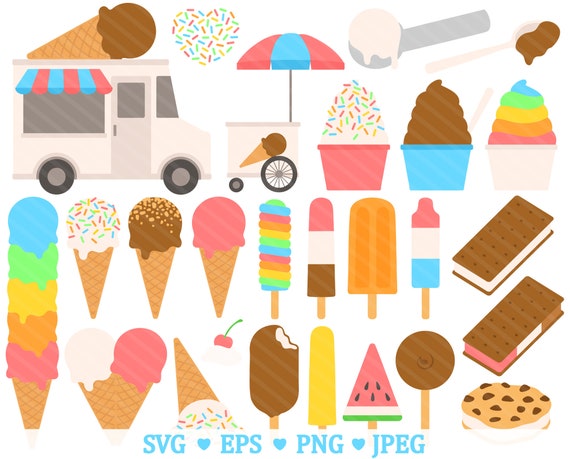This vibrant and colorful digital illustration features an array of various cold treats in a simplistic, minimalist style. The flat design emphasizes the multitude of ice cream-related delights, with no attempt to give a 3D perspective, except for a few detailed ice cream sandwiches. The top left corner showcases a white ice cream truck adorned with a pink and blue striped awning and a giant chocolate ice cream cone on its roof. Nearby, an ice cream cart equipped with large front wheels, small back wheels, and a multicolored umbrella stands out. Scattered throughout the image are numerous ice cream cones, featuring a spectrum of toppings in shades of blue, green, pink, brown, and yellow. Some cones are adorned with sprinkles, including a particularly tall cone with five layers of ice cream in pink, orange, yellow, green, and blue. Various popsicles are also depicted, including classic bomb pops, a colorful swirly popsicle, and a frozen watermelon slice. Ice cream cups fill the top right section, showcasing multicolored scoops in sundae dishes, with one cup displaying a delightful mix of sprinkles. On the bottom right sits a cookie-style ice cream sandwich, complete with chocolate chip cookies sandwiching vanilla ice cream. Text in blue at the bottom of the image states "SVG part, EPS part, PNG part, JPEG," indicating the image's versatility in different digital file formats.